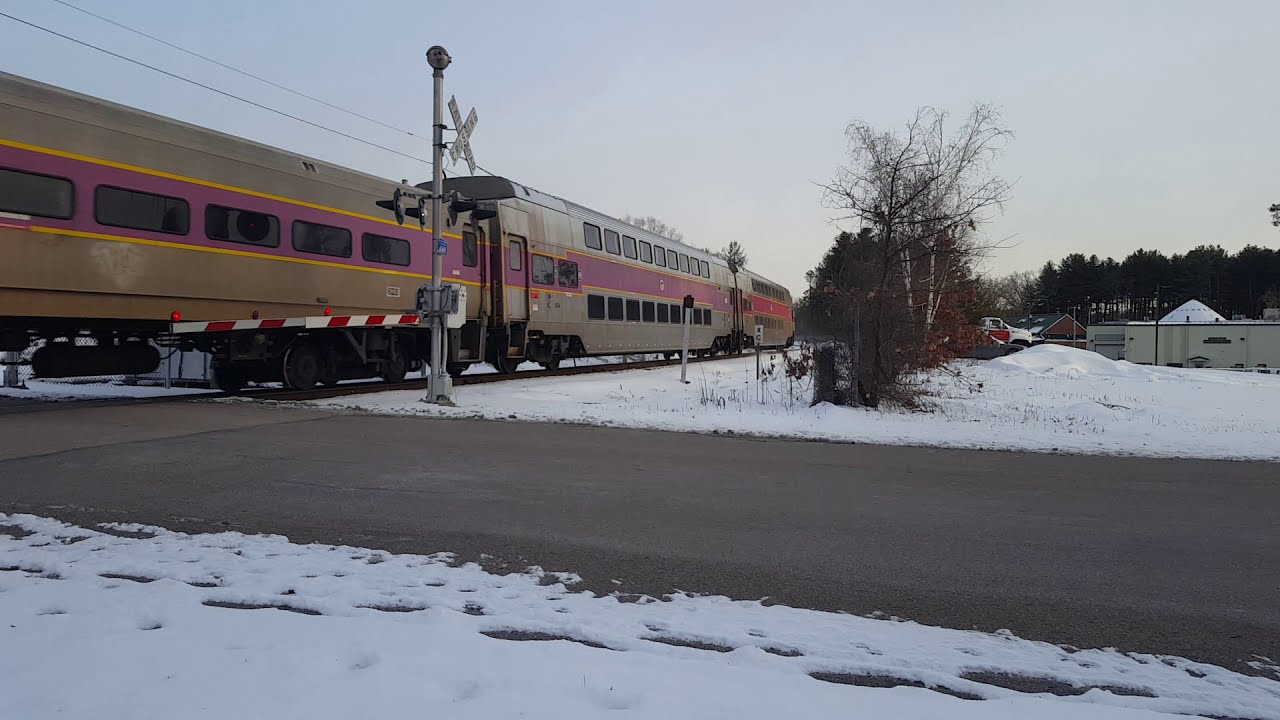In this color photograph, taken during a cloudy, overcast day, we see a detailed scene of a train crossing a road. The road runs horizontally across the image, intersecting with the railroad tracks. The train, which appears from the left side of the picture and disappears into the distance at the center of the frame, is striking with its bronze or silver body. Distinguishing the train are purple stripes surrounding the windows, accentuated by gold or yellow stripes above and below. The train is identified as a passenger train, with small windows running along its side. A prominent feature is the lowered white and red striped railroad crossing gate, equipped with round red reflectors, blocking any non-existent cars from passing. The scene is blanketed in about two inches of white snow, covering the grass on either side of the road. In the background, we see some leafless trees, as well as a few evergreen trees, and a couple of buildings towards the right side of the image. The sky overhead is a grayish-blue, typical of a cloudy day.